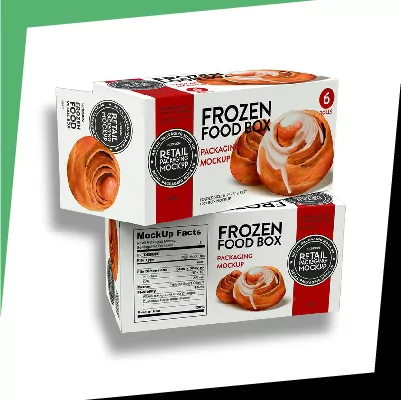The image shows a carefully designed mock-up for frozen cinnamon rolls, set against a predominantly white background with artistic elements. The upper left corner features a green triangular frame that thickens towards the corner and tapers off both horizontally and vertically. Similarly, the lower right corner has a black triangular frame. In the center of the image, there are two identical boxes of cinnamon rolls—one displaying the front and the other showcasing the back. The front box prominently presents the label "Frozen Food Box" in large black capital letters, accompanied by a smaller red text that likely reads "Packaging Mock-Up." A striking image of two cinnamon rolls with dripping icing is also featured, along with a red circular label that seems to indicate the number "6." On the top left of the front box, there is a horizontal red strip with a black circular emblem containing additional white lettering. The bottom box mirrors the first but shows the back side, complete with "Mock-Up Facts" and the same emblematic features as the front. The entire image has a sleek, modern appeal, potentially intended for an advertisement or promotional poster.